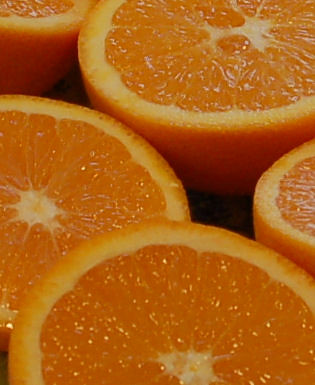This close-up shot captures five halves of ripe oranges that have been cut in half and are tightly packed together. The image is highly detailed, showing the glistening, juicy flesh of the orange segments and the pith underneath the pale orange rind. The bright orange color of the fruit contrasts with its white center and starburst-like core. The cut halves are all facing upwards, positioned haphazardly and overlapping one another on a dark, possibly greenish or brown, background. This high-quality, professional photograph focuses on the freshness and juiciness of the oranges, making them look exceptionally ripe and delicious.